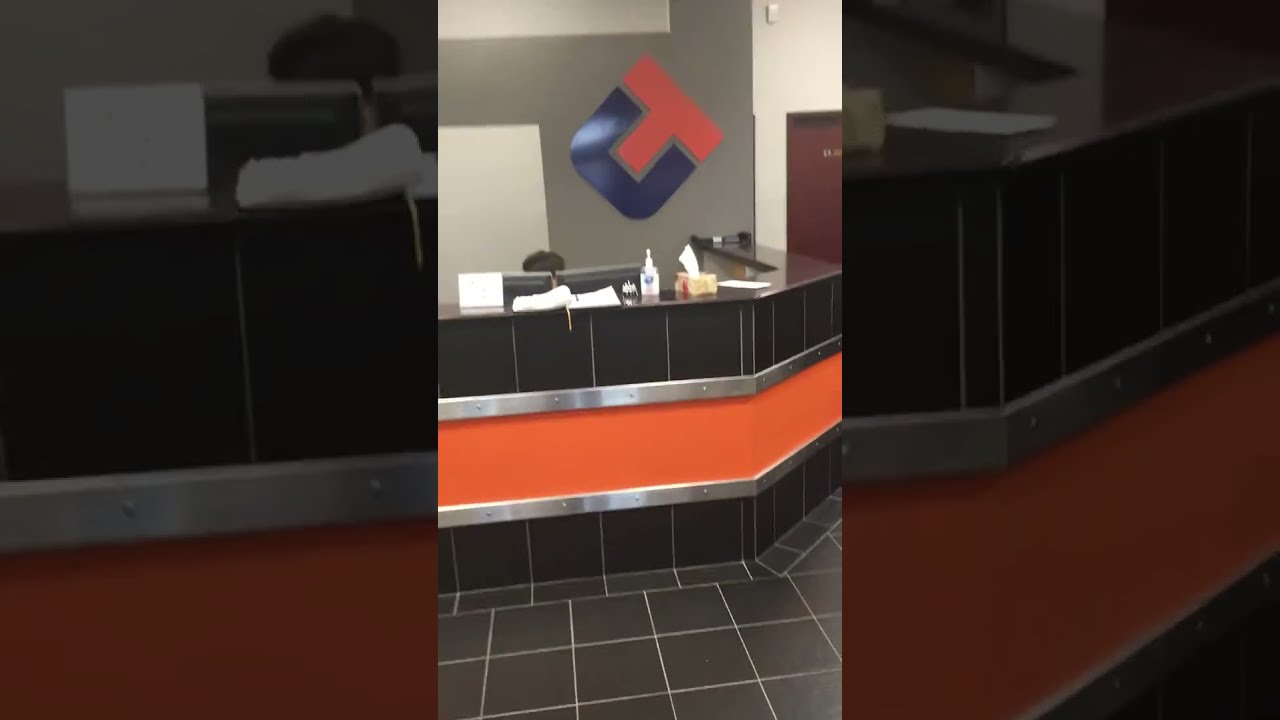The image depicts a reception desk situated in the middle of the frame, flanked by two vertical black rectangles on the left and right sides. The desk, potentially part of a lobby or bank, features a prominent horizontal orange stripe on its exterior, which is adorned with black tiling that extends down to the tiled floor. On the counter, there is a neatly arranged assortment of items including hand sanitizer, a box of Kleenex, a bell, and an open binder. Behind this desk, two computer screens are visible along with the dark hair of a receptionist. The wall behind the desk is partly gray and features a black and red logo, which might represent a navy 'C' interlocked with an orange 'T' or possibly the letters T and U. To the right of the desk, a partially visible brown door hints at another section of the building, potentially a bathroom. The floor in front of the desk is made up of black tiles separated by white grout lines.